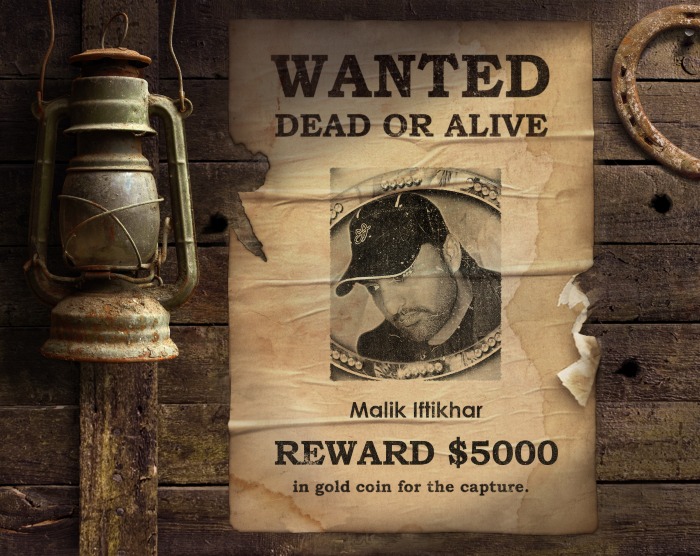The image depicts a graphic design reminiscent of an old Western wanted poster, prominently displayed against a backdrop of weathered, horizontal wooden boards that evoke the feel of a barn or fence. At the center of the scene is the tattered and stained poster itself, rendered on cream-colored paper that bears the marks of time with rips and tears primarily at the top left and center right edges. Bold black letters at the top of the poster declare "WANTED," followed by "DEAD OR ALIVE." The monochromatic photograph in the middle shows a man wearing a black baseball cap with a white-bordered bill. The man, with a light, unshaven beard and dark hair, looks down towards the lower-left corner of the poster, his exact expression obscured by shadows. He is dressed in a dark garment, either a shirt or a jacket, difficult to discern amid the grayscale aesthetic. Below his image, the name "Malik Iftikhar" stands out, followed by the promise of a $5,000 reward in bold black letters, with further clarification in smaller script below that this bounty is payable "in gold coin for the capture." Adjacent to the poster, an old, rusted horseshoe is affixed to the upper right via an aged nail, while an antiquated gas lamp—alluded to be an antique—hangs to the left, its dusty, light-green body suggesting it's long lost its function. Both the horseshoe and the lamp add to the historical ambiance, anchoring the poster in a tableau that blends graphic design with nostalgic elements of antiquity.